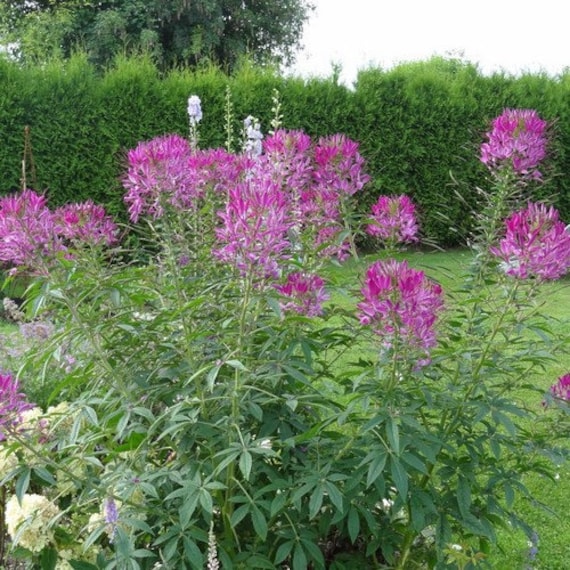This image captures an outdoor garden scene dominated by tall, slender-stemmed flowers with long, skinny green leaves. The flowers, predominantly in vibrant shades of lavender and pinkish-purple, stand tall in the forefront, with clusters extending from the left to the right of the frame. Among them, a few white flowers—possibly hydrangeas—pepper the lower corners of the image, adding contrast. In the background, a row of unruly green shrubs and several large trees with lush green leaves frame the scene, beneath a cloudy, white sky that suggests an overcast day. The grass throughout is short and verdantly green, completing this lush and colorful pastoral setting.